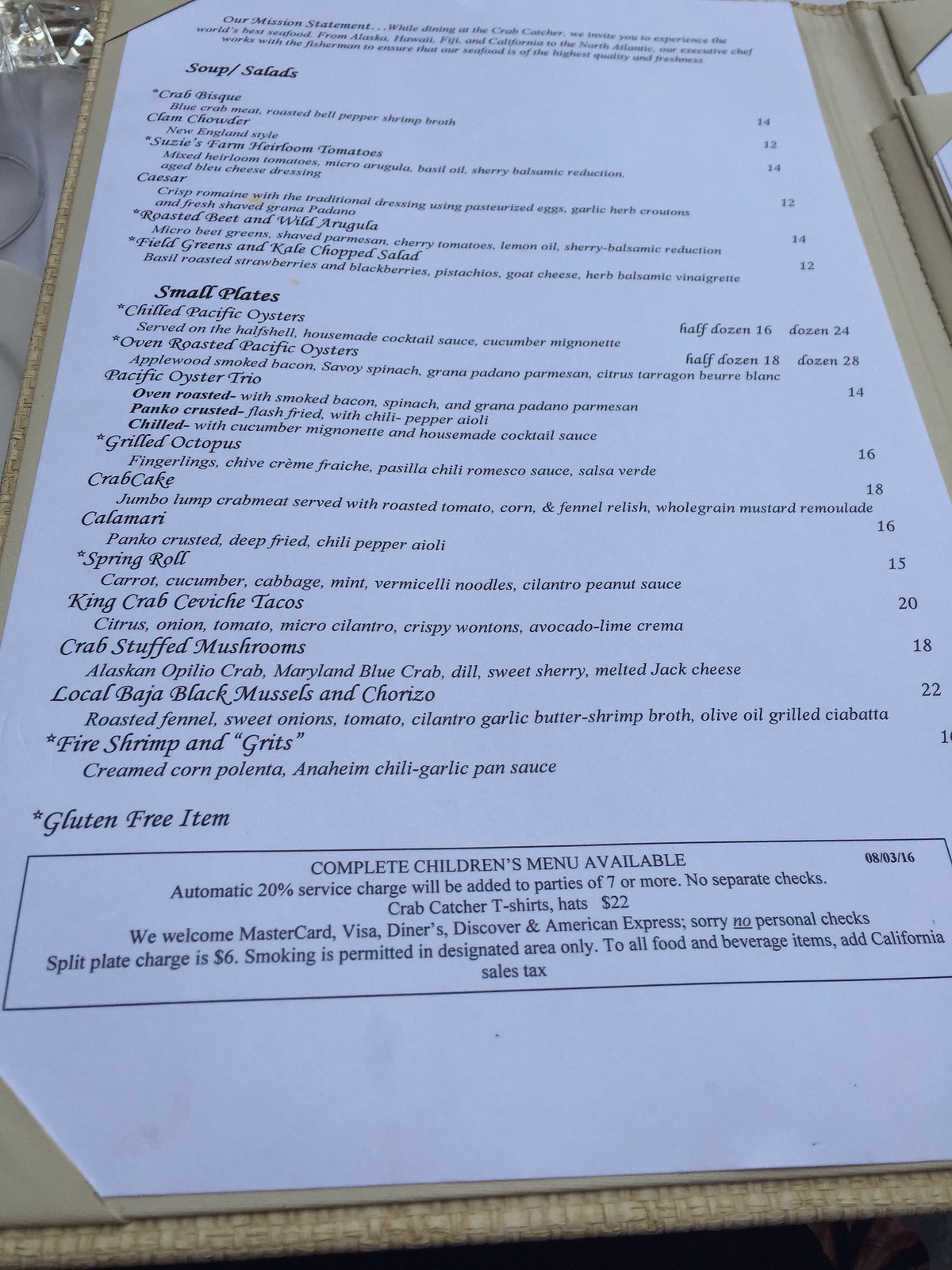The photograph offers a detailed, angled view of an open menu inside a TAM binder, with the perspective looking down at the inside of the back cover. The page is white, featuring a two-column layout: meal descriptions on the left and prices on the right. 

At the very top of the page, a blurred mission statement is partially visible. Below it, the heading "Soup/Salads" is prominently displayed in black text, followed by five or six lines listing various salad options.

The subsequent subheading reads "Small Plates," and the text becomes clearer, detailing seven or eight dishes starting with "Chili Pacific Oyster" and followed by "Oven Roasted Pacific Oyster," among others. 

An asterisk at the bottom indicates gluten-free items, and there's a rectangular block with information about a complete children's menu. 

In the upper left corner of the image, a portion of a white tablecloth and a water-filled drinking glass are visible, while the upper right corner shows the inside fold of the menu, appearing white and presumably the other side of the menu.

The image is well-focused, though dimly lit, and the menu itself appears clean and well-maintained.